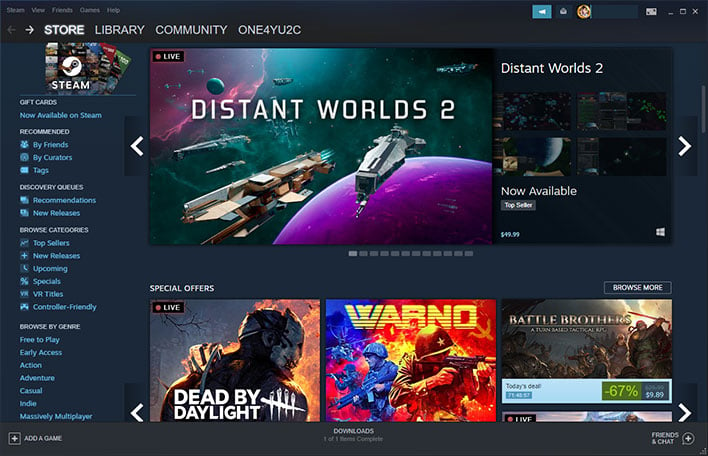A screenshot captured from the Steam app on a computer. At the top, a black navigation bar displays links for 'Steam', 'View', 'Friends', 'Custom Games', and 'Help'. Below this, another set of links includes 'Store', 'Library', 'Community', and 'U2C'. On the left side, a promotional image for Steam gift cards is visible alongside various categories including 'Now Available on Steam', 'Recommended by Friends', 'Curators and Tags', 'Discovery Cues', 'Recommendations', 'New Releases', 'Browse Categories', 'Top Sellers', 'Upcoming', 'Specials', 'VR Titles', and 'Controller Friendly'. Further down, users can browse by genre with options for 'Free to Play', 'Early Access', 'Action', 'Adventure', 'Casual', 'Indie', and 'Massively Multiplayer'. The central section showcases the current storefront with a highlighted image of the game 'Distant Worlds 2' and additional clickable thumbnails for more featured games. Below this, a 'Special Offers' section lists games like 'Dead by Daylight', 'Warno', and 'Battle Brothers', allowing users to click for more details, reviews, images, and gameplay videos, or proceed to purchase.